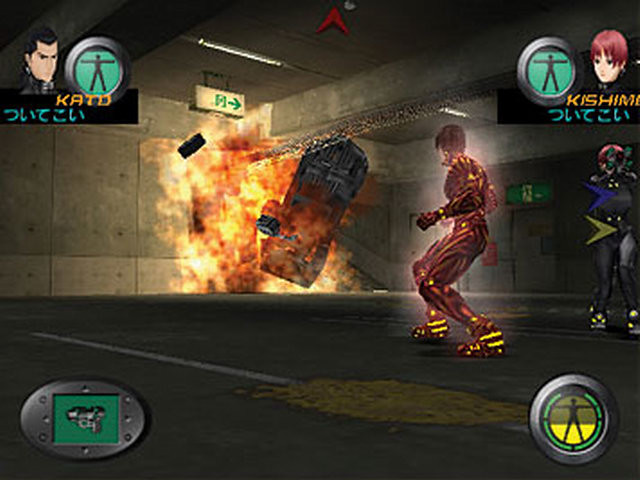In this gameplay screenshot, two character names are partially visible at the top of the screen: a male character labeled "K-A-T-D" and a female character labeled "K-I-S-H-I-M." The man is depicted alongside a woman with striking red hair. In the dynamic action below, a character dressed in a red and yellow suit occupies the foreground, with a dramatic car explosion occurring in the background. Near the bottom of the screen, another character appears with their arms fully extended, seemingly exhausted as their energy bar, displayed in yellow, depletes down to their knees. The scene is filled with intense action and vibrant colors, capturing a moment of high-stakes drama within the game.